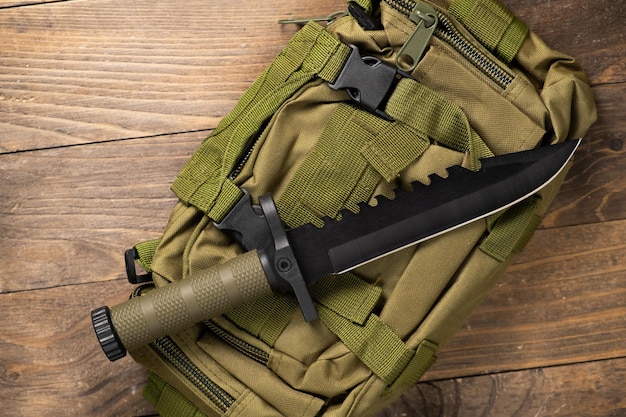This photograph captures a meticulously detailed view of an army green canvas bag, centrally placed on a medium brown, grained wooden floor or table. The bag, which appears to be a compact pouch rather than a full-sized backpack, features darker shades of green on its flaps and straps. It is adorned with heavy, woven straps and black buckles, indicative of rugged, outdoor gear, and includes two zippered sections—one likely opening the main compartment and another on an exterior pocket.

Prominently displayed on top of the bag is a large, distinctive knife. The knife, suited either for a soldier or an outdoor enthusiast, boasts a black, jagged blade designed for sawing as well as cutting. Its grip, army green with small nubs for enhanced hold, extends to a ridged, black circular bottom. The knife's detailed design and robust construction suggest it is a reliable tool for various demanding tasks. The overall scene radiates a sense of readiness and adventure, emphasizing the utility and newness of both the pouch and the knife.